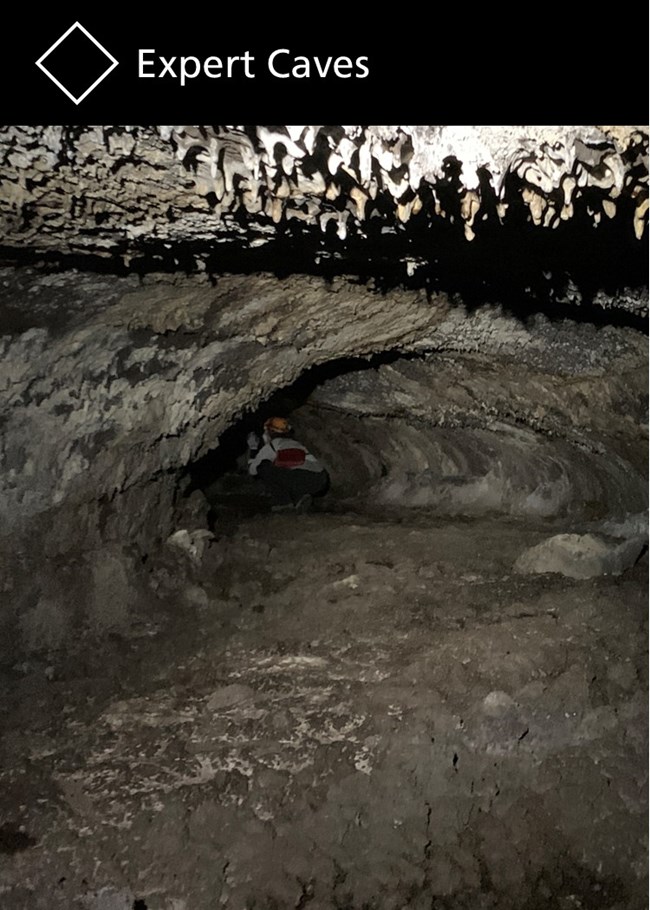The vertical rectangular image features a black border at the top with a white diamond shape and the text "Expert Caves" to its right. Below this, the photograph depicts the entrance to a cave, showcasing a rough, textured cave ceiling adorned with stalactites. The cave wall is predominantly gray and rugged. In the center of the image, there's a small arched entryway leading deeper into the cave, which extends back and curves to the left. The foreground shows rocky, gray ground broadening out toward the viewer.

A person is seen crouched down to fit through the small archway. They are dressed in jeans, a long-sleeve white shirt, and a hard hat, which seems to be orange. They carry a red bag on their back and hold something out in front of them. The dark shadows on the right side contrast with the brown, beige, and gray hues of the cave material, composing the overall rugged yet intriguing scene of exploration.